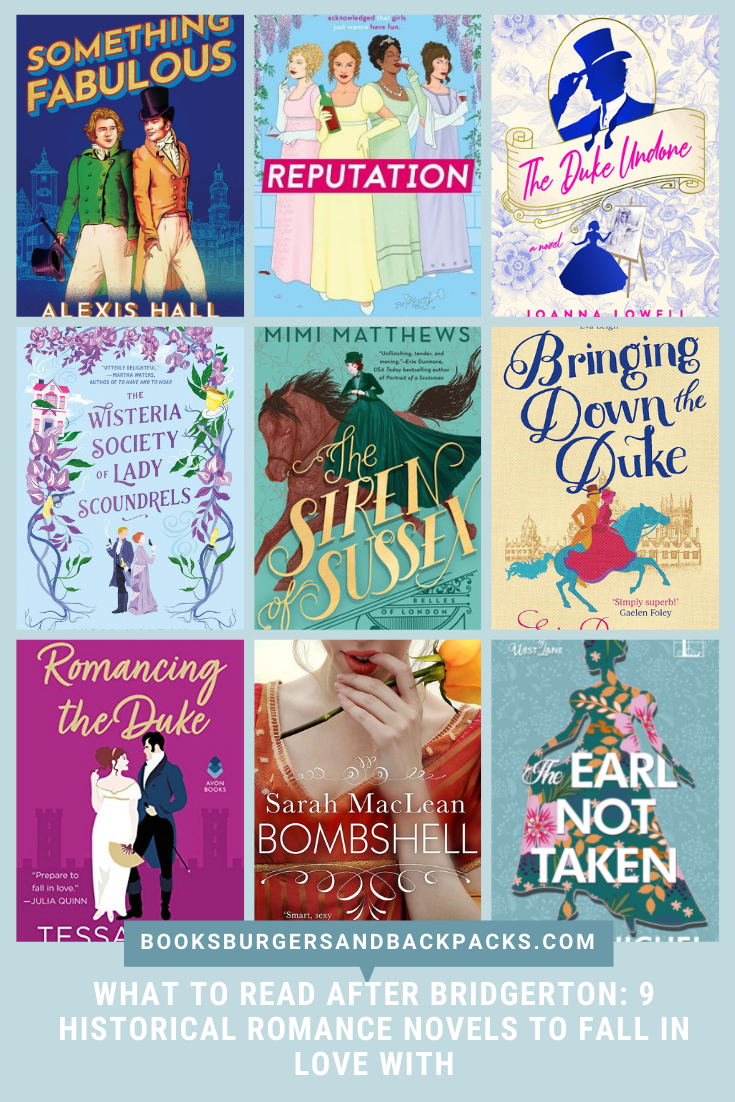The image is a vibrant and colorful poster featuring a grid of nine historical romance novel covers, arranged in three rows and three columns. Each cover is distinctive in design, showcasing rich hues like purple, blue, green, pink, yellow, and teal.

**Top Row (Left to Right):**
1. **Something Fabulous** by Alexis Hall - Features two men leaning against each other, with one wearing a top hat.
2. **Reputation** - Depicts four women enjoying drinks together.
3. **The Duke Undone** - Shows a silhouette of a person in a top hat.

**Middle Row (Left to Right):**
4. **The Wisteria Society of Lady Scoundrels** - Illustrates a man and woman.
5. **The Siren Sussex** - Features a woman riding a horse.
6. **Bringing Down the Duke** - Shows a man and a woman riding a horse together.

**Bottom Row (Left to Right):**
7. **Romancing the Duke** - Depicts a man and a woman gazing at each other romantically.
8. **Bombshell** by Sarah McLean - Shows a woman seductively biting her finger.
9. **The Earl Not Taken** - Features a silhouette of a dancing woman.

Across the lower bottom of the poster, in white capital letters against a blue bar backdrop, it reads: "BooksBurgersAndBackpacks.com" and "What to Read After Bridgerton: Nine Historical Romance Novels to Fall in Love With." The overall design suggests it's an advertisement aimed at fans of historical romance novels, encouraging readers to explore these captivating stories.